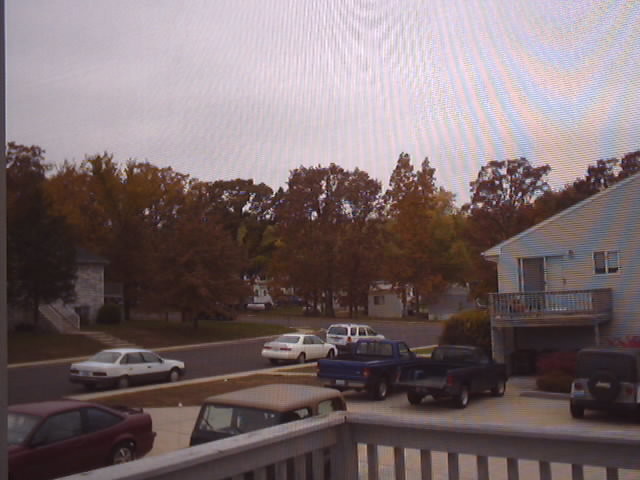The color photograph appears to have been taken from an upper deck of a house, possibly through a screen door or an electronic display like a CCTV screen, as evidenced by the warping swirls and undulating stripy lines particularly visible in the top right corner. The scene depicts a suburban neighborhood. The focal point is a residential street lined with multiple houses and large trees adorned with brown leaves, hinting at the autumn or early winter season. 

In the foreground, several cars are parked: a maroon car, a jeep-like vehicle with a black upper part and silver bottom, and two trucks. Among the vehicles, a sequence of three white cars appears to be aligned along the road, heading towards the right side of the frame. Across the street, the neighboring houses mirror the upper deck and handrail design, with one house notably featuring a small balcony with a greyscale exit door. Between the street and the houses on the near side, there is a grass verge. Additionally, the background reveals more houses with balconies and a parking area filled with dark-colored trucks, one of which is noticeably a jeep. The street layout and the arrangement of cars and houses contribute to a scenic view of this tranquil residential area.